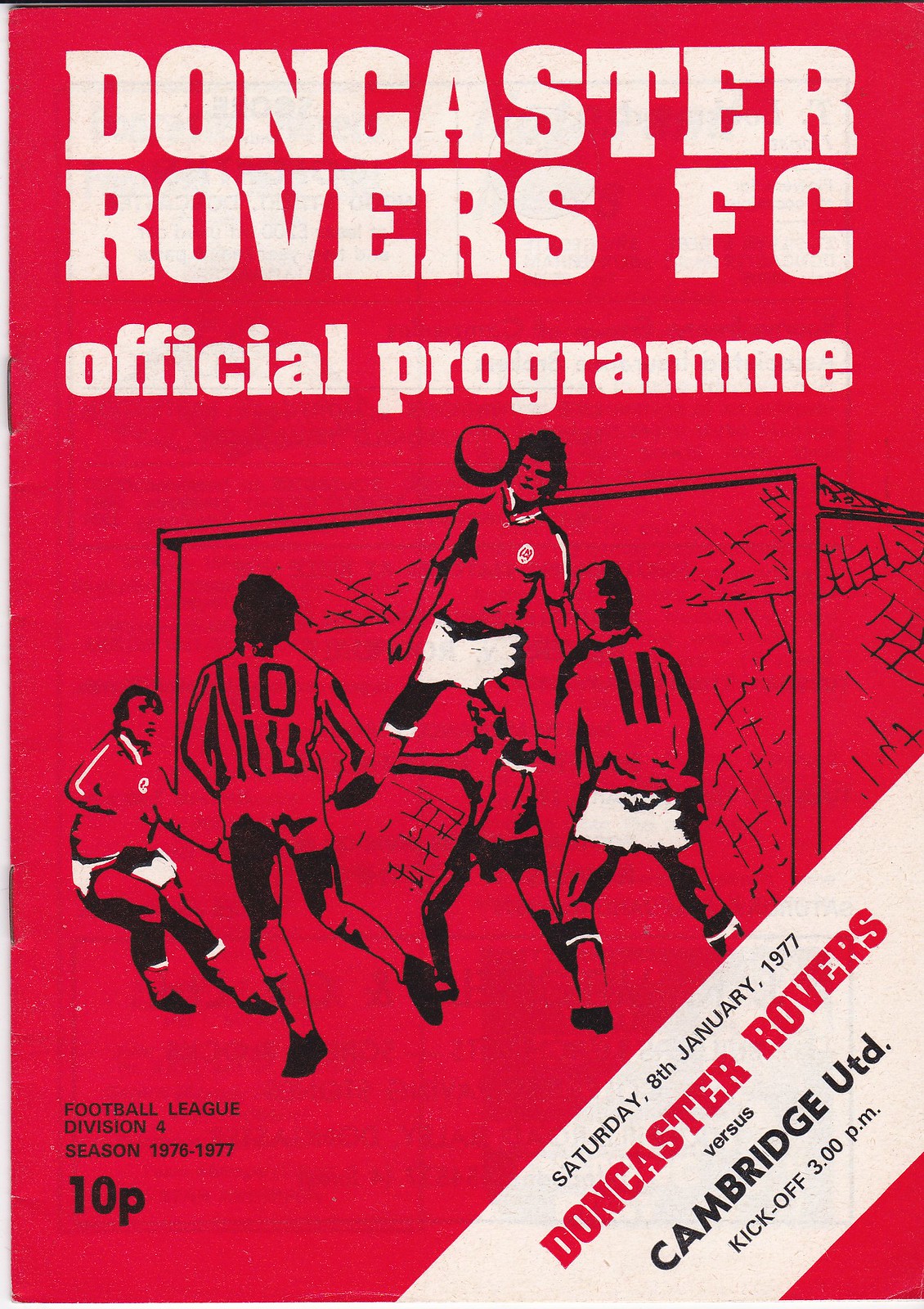This image showcases an official program cover for Doncaster Rovers FC, set against a solid red background. Dominating the top third in large white text are the words "Doncaster Rovers FC" followed by "Official Program." The illustration beneath this header depicts a dynamic soccer scene: a player in midair appears to head the ball near the goal net, with the goalie in action and three other players—two with numbers 10 and 11 on their jerseys, their backs turned—participating in the game. The image is predominantly rendered in red, black, and white, with players' shorts and some shirt stripes highlighted in white. Black text at the bottom left corner states "Football League Division 4 Season 1976-1977, 10-P," indicating the program's price. Additionally, a diagonal white stripe runs from the bottom center to the right, inscribed with "Saturday 8th, January 1977" in black text, "Doncaster Rovers" in red, "Versus" in black, "Cambridge UTD" in black, and the kickoff time "3-0-0-P-M" in black.